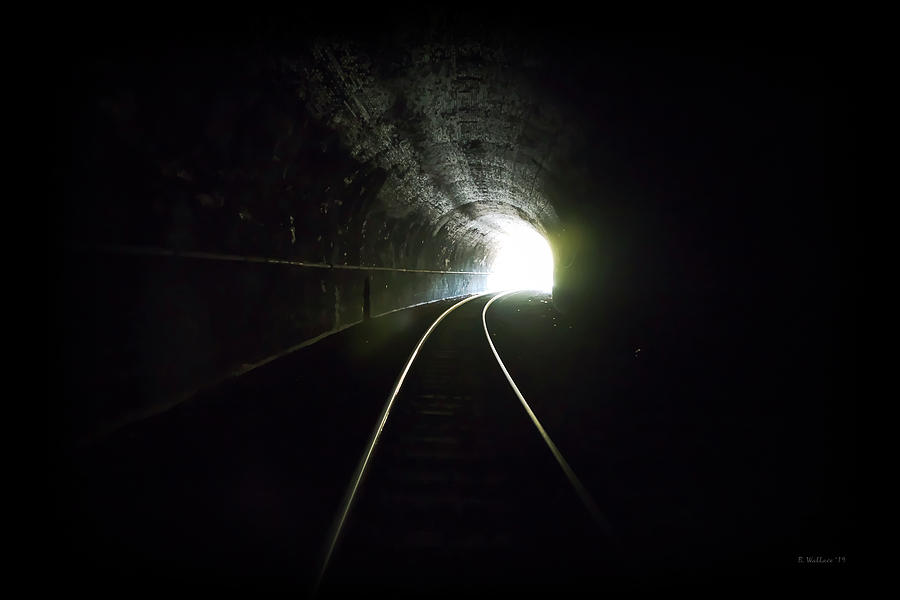The image depicts a dimly lit train tunnel, where a bright light at the far exit illuminates the otherwise dark, cavernous passage. The polished, silver-colored train tracks at the bottom of the picture reflect this incoming light, enhancing their visibility against the surrounding shadows. The stone walls of the arched tunnel curve elegantly, catching subtle reflections that hint at their rough, circular structure. This light not only serves as a beacon but also casts soft rays that stretch towards the viewer, creating a stark contrast between the darkness and the luminescence. In the lower right corner of the image, there's a faint watermark, possibly reading the name "E. Williams" or "E. Wallace," indicating it might be the artist or photographer's signature. This scene conveys both the isolation within the dark tunnel and the hopeful promise of emerging into brightness.